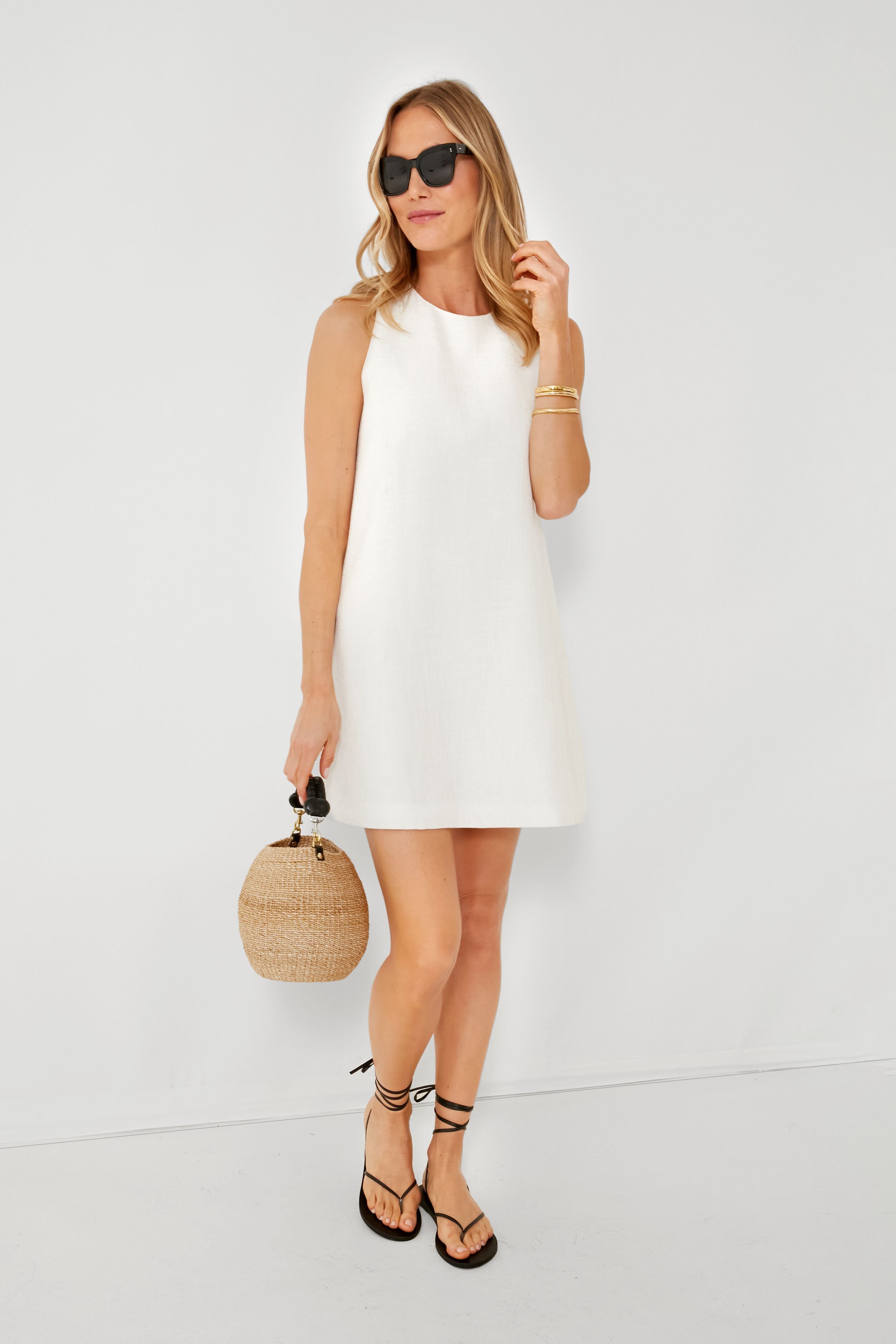The photograph features an attractive Caucasian woman with a fair complexion, standing against a white wall and floor, likely in a studio setting for a photo shoot. She appears to be in her late 20s to early 30s and has mid-length, blonde hair with highlighted strands that transition from dark blonde to a lighter brownish shade. Her hair cascades below her shoulders, and she is wearing black, oversized designer sunglasses that obscure much of the top part of her face.

Her outfit consists of a simple, sleeveless white dress that reaches down to about her mid-thigh, leaving her legs exposed. She complements this attire with black, ballet-style shoes that function like sandals at the bottom but feature ties that wrap around her ankles in a ribbon-like fashion. Her feet are bare, without any nail polish.

In her right hand, she carries a unique, tan wicker-like designer bag, which appears handcrafted with a crocheted style. The bag is rounded and features a black leather handle attached with gold chains at the corners. Her left hand is raised, touching her hair, and on her wrist, she wears three thin, gold bracelets—two stacked closely together and one positioned slightly higher on her forearm. Her lips are painted in a neutral, nude-pinkish blush color, adding to her understated elegance.

Overall, the image captures her poised stance and subtle details, emphasizing her fashionable, yet minimalistic, style.